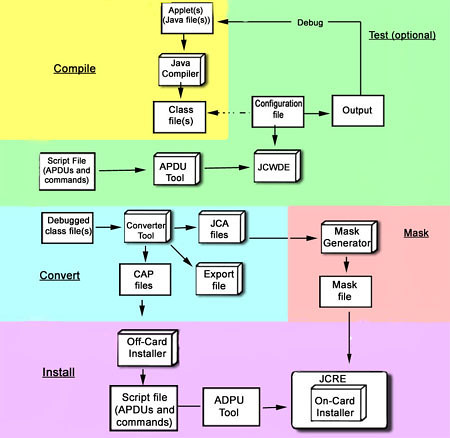The image is a detailed flowchart for a computer programming process, featuring five distinct sections colored yellow, green, peach, turquoise, and purple. It begins at the top left with a yellow box labeled "Compile" and follows a clockwise direction. Each main box contains smaller white boxes with black text and arrows indicating the flow. Starting from "Compile," there's a sequence of white boxes: "Applets, Java files" leading to "Java Compiler," and then to "Class Files." A light blue box labeled "Debug" is interspersed, pointing back to "Applets, Java files." Adjacent to the Compile sequence is the green section labeled "Test Optional," which connects to a white box labeled "Output" and another labeled "Configuration File." Continuing clockwise, the next section is a peach-colored box labeled "Mask," followed by a turquoise box labeled "Convert," and culminating with a purple box at the bottom labeled "Install." The entire flowchart consists of about 20 interconnected white boxes arranged within these five colorful sections, detailing a comprehensive overview of different stages in the programming workflow.